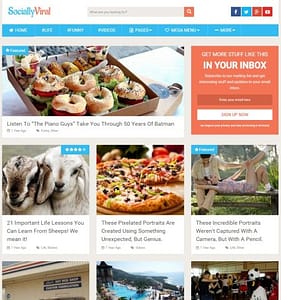A colorful assortment of bagels displayed on a tray, accompanied by an eclectic gathering: two goats browsing nearby, a partially eaten pizza with one slice missing, people sharing an intimate moment on a park bench, a quaint house with a swimming pool in the background, and a whimsical panda bear curiously situated inside a restaurant-themed mailbox.